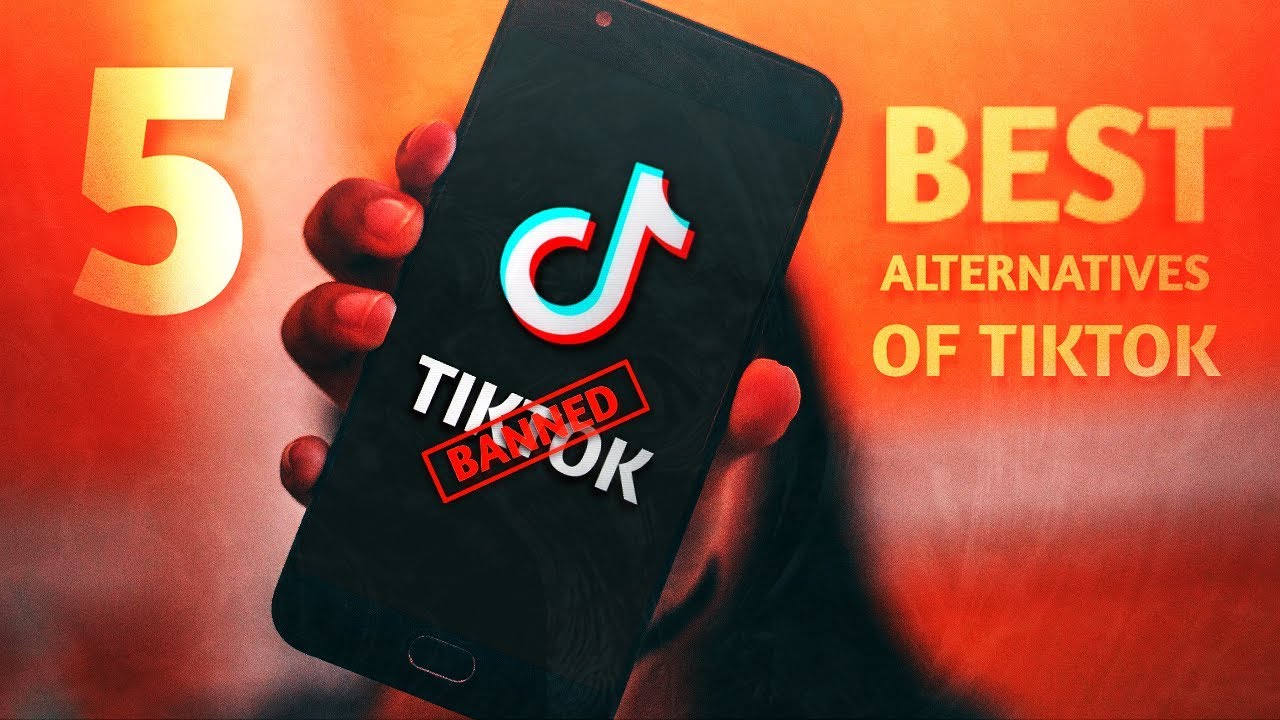The image features a right hand holding a navy smartphone, pointing it outward. The smartphone screen displays the text "TikTok Banned" in white lettering. Adjacent to the text is the TikTok logo, which is composed of green, white, and red colors. Superimposed on the phone screen is a red "Banned" stamp.

The background of the image transitions from a vibrant red at the top to a darker, grainier shade at the bottom, creating an intense atmosphere. On the left side of the image, in yellow text, it reads "5 Best Alternatives." The overall visual is an advertisement promoting alternative apps, suggesting options due to the banning of TikTok.